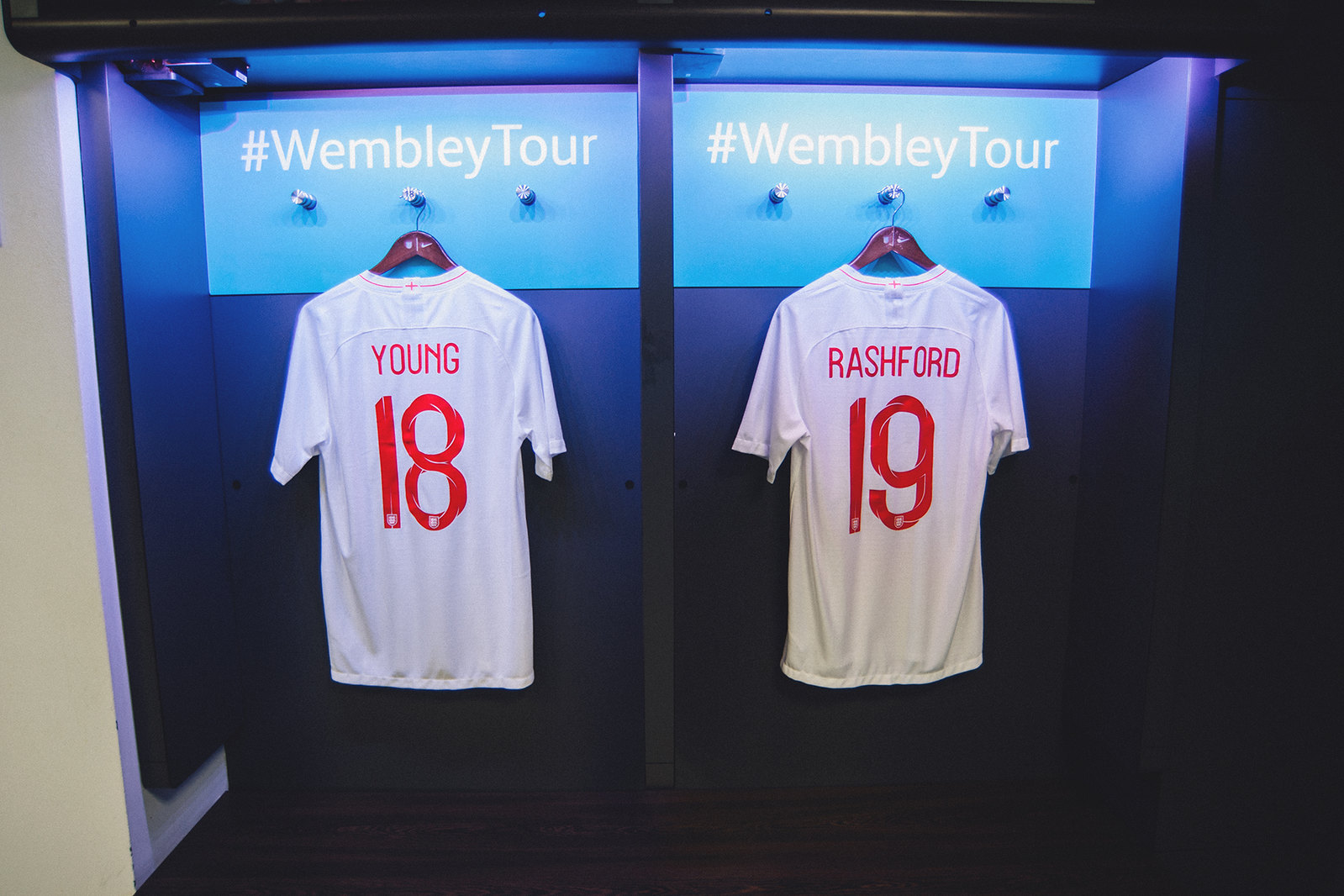You are looking at an installation that appears to be a sports locker room setup, specifically styled for a presentation or tour display. The wall is predominantly dark blue, fading to black towards the bottom, with illuminated light blue sections at the top that highlight the reflective banners reading "#WembleyTour" in white, sans-serif font.

The display features two enclosures, resembling shallow stalls, each outfitted with three pegs for hanging items. In each stall, the middle peg holds a wooden hanger with an immaculate white team jersey. 

The jersey on the left bears the name "YOUNG" in bold red, sans-serif lettering, with the number "18" prominently displayed below it in a custom stylized font. Similarly, the jersey on the right reads "RASHFORD" in the same bold red lettering, with the number "19" printed large beneath it.

The white jerseys also have red seams around the collars, adding a touch of detailing to their design. The overall illumination of the stall creates a purplish glow, enhancing the visibility and creating a visually striking display.